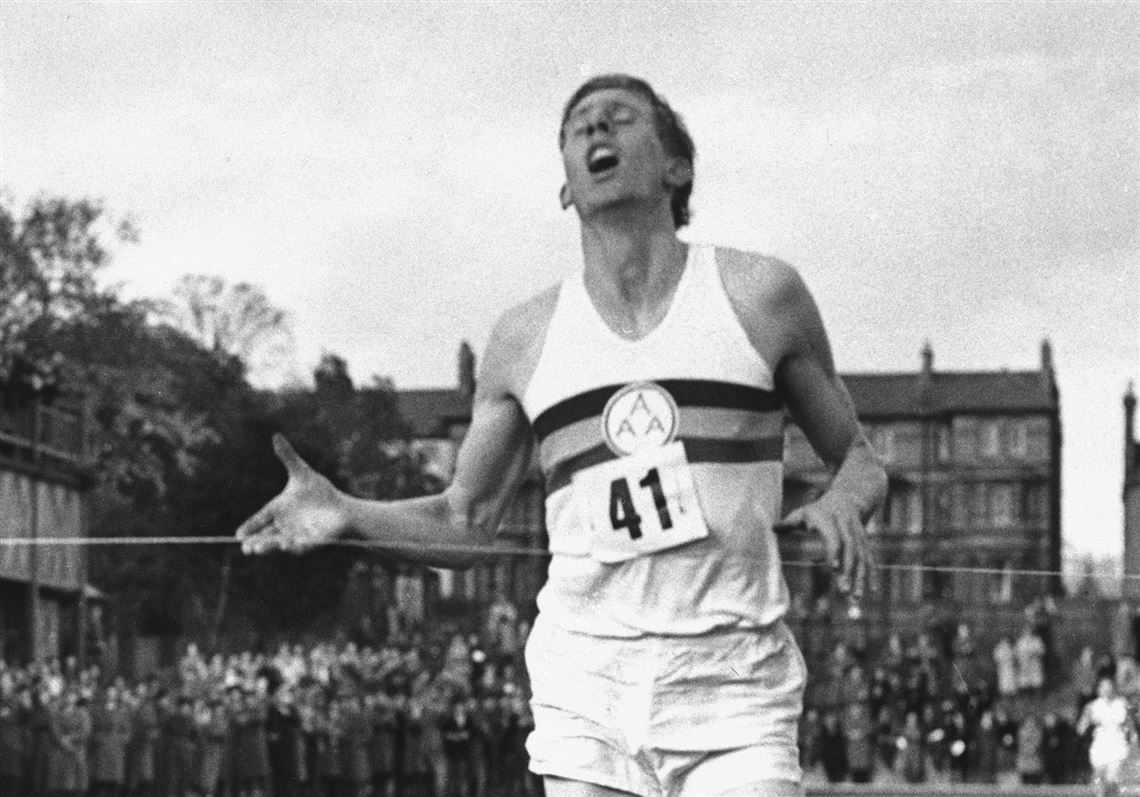This is a vintage black-and-white photograph captured outdoors in horizontal landscape orientation, featuring the historic moment when runner Roger Bannister crosses the finish line in a foot race around 1954. The subject, a man photographed in a medium crop, is wearing a white tank top with a black and gray stripe across the chest and shorts, with a number placard displaying '41' pinned to his jersey. He appears to be in motion, indicated by his outstretched hands beside him and his mouth open in a relieved expression with his eyes closed, likely signifying the intense effort exerted. Behind him, a large crowd of spectators is gathered, watching intently, with multi-story buildings providing an urban backdrop, suggesting the race is taking place in a city setting. The overcast sky inferred by the grayscale adds a dramatic tone to this momentous image of athletic achievement.